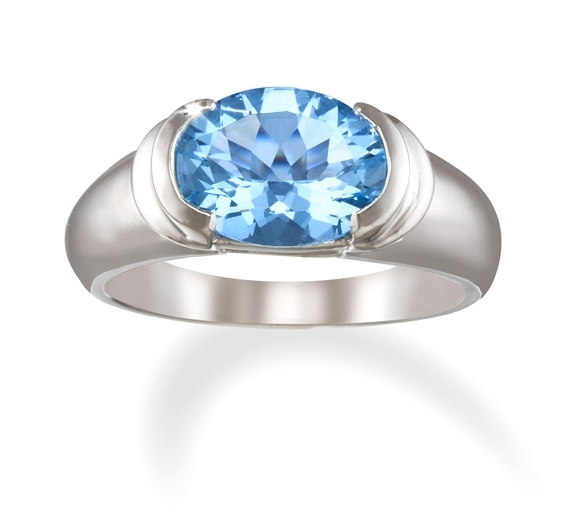This highly detailed and close-up image, possibly a photograph or a computer-rendered illustration, showcases a silver-toned ring with a thick band, either of sterling silver, white gold, or platinum, displayed against a stark white background. The ring features a large, oval-shaped, light blue gemstone, likely a sapphire, topaz, or aquamarine, characterized by its multifaceted, sparkling surface that catches the light beautifully. The gemstone is set securely into the band with a metallic silver bezel that holds it in place on either side. The ring has a simple, smooth, and possibly matte finish with no additional adornments, except for the bezel design which hugs the gemstone, adding depth and interest. The image gives a sense of the ring standing upright, casting a light gray shadow on its white surface, emphasizing the ring's form and the stone’s brilliance.